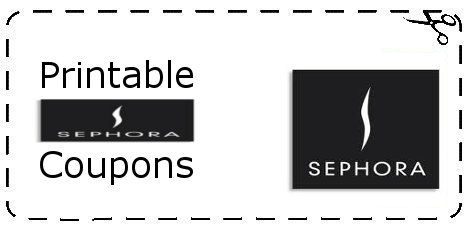The image features a black, dashed line forming a rectangular border in the upper right corner. Inside this border, there's an illustration of a pair of black scissors, suggesting a cut-out coupon. On the left side, the word "printable" is prominently displayed. Adjacent to it, a black bar features a white "S" logo, followed by the word "Sephora" in bold, both in white typography. Below these elements, the word "coupons" appears in black text. On the right side of the image, there's a larger black box with the same stylized "S" logo and the word "Sephora" within it. The background of the image is plain, ensuring that the text and icons stand out clearly.